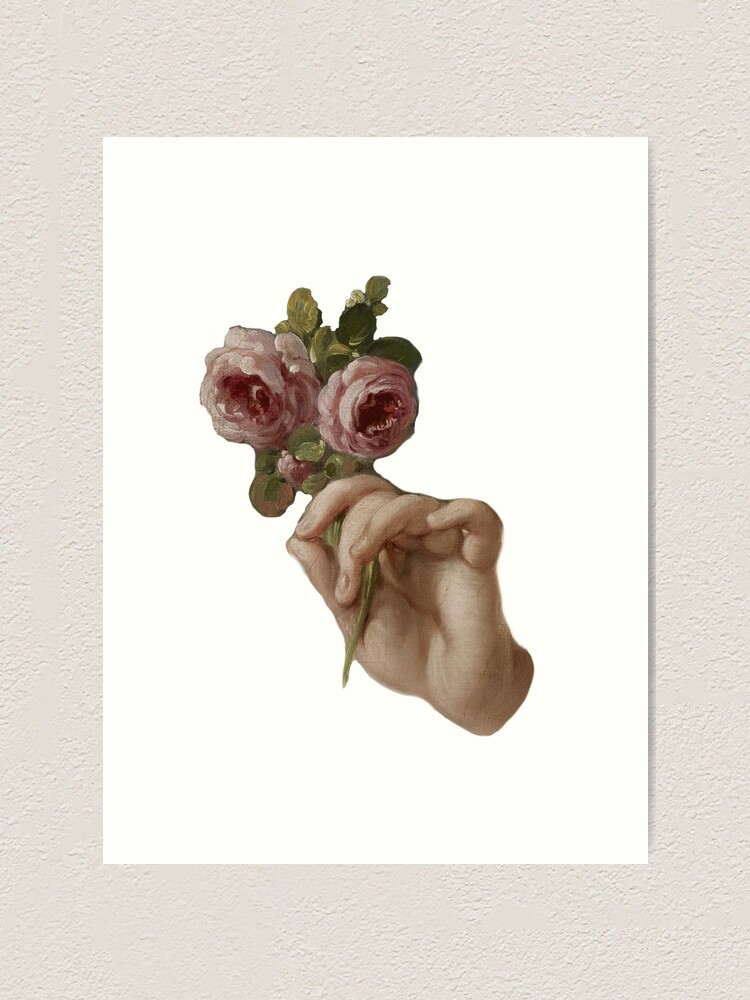The image showcases a detailed painting mounted on a textured, beige wall. The centerpiece of the painting is a brownish-hued hand, resembling that of a female, depicted clasping a stem with blooming flowers. The hand's grasp is unique, creating a circle with the thumb and index finger around the stem. The stem bears three flowers of varying sizes, with petals in shades of pink to light pink, and some petals subtly transitioning to red. Green leaves accompany the flowers, which are notably without thorns. The artwork, executed in a watercolor style, appears on a white sheet, emphasizing the vibrant colors and delicate floral theme against the minimalist background.